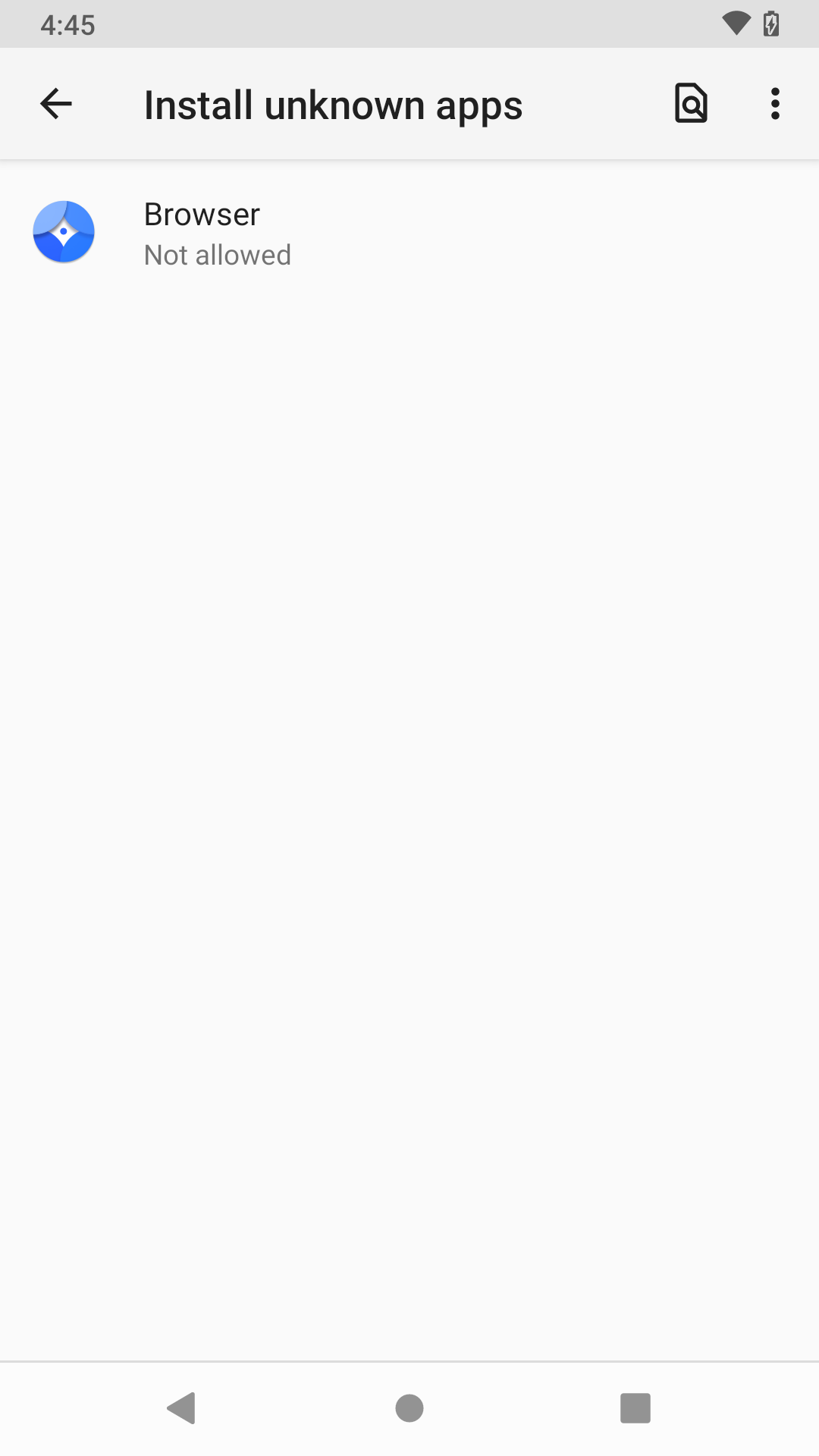This is a detailed screenshot from a smartphone device. At the top, there is a dark gray status bar displaying the time "4:45," along with icons for Wi-Fi and battery status, the latter indicating a very low battery level. Below this, a lighter gray navigation bar features a black back arrow and the label "Install Unknown Apps." This bar also includes an icon resembling a piece of paper with a magnifying glass and, on the far right, a vertical trio of black dots.

The main section of the screenshot prominently displays a blue circle with a white diamond shape in its center, which encloses a smaller blue circle. This graphic is accompanied by the text "Browser Not Allowed." At the bottom of the image, a navigation bar presents a gray back arrow, a gray circle, and a gray square.

The image is purely graphical with no photographic content, and contains no depictions of people, animals, birds, plants, flowers, trees, buildings, bridges, signs, or billboards.